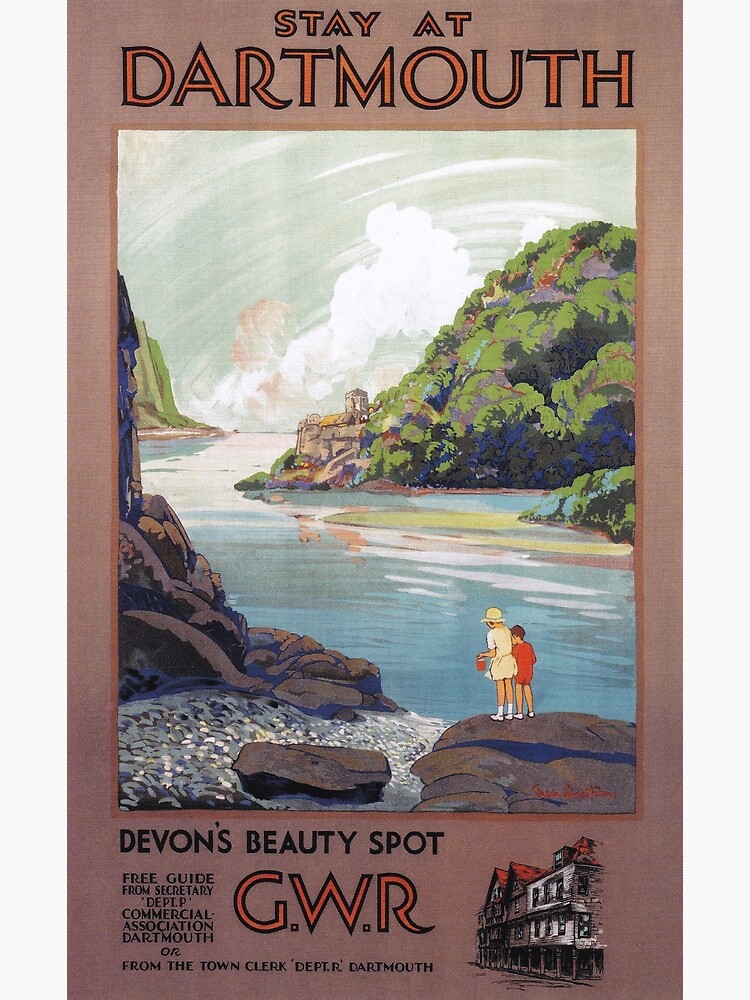This detailed tourism poster, reminiscent of the 1920s or 1930s, features a captivating brownish background with vivid orange font outlined in black at the top reading, "Stay at Dartmouth." Central to the poster is a painting encased in a light brown border, illustrating a serene outdoor scene. The painting showcases a meandering river flanked by lush green hills on the right and rocky hills on the left, where a woman in a white dress and yellow hat stands beside a child dressed in a red shirt and shorts. Below the painting, "Devon's Beauty Spot" is prominently printed in black. Secondarily, the poster includes "GWR" in orange font similarly outlined in black. Adjacent to this, on the left, pertinent information about acquiring free guides from the Secretary Department Commercial Association or the Town Clerk Department in Dartmouth is clearly provided in black font. Adding to the charm, a small image of brown and white row houses with red roofs appears at the bottom right.